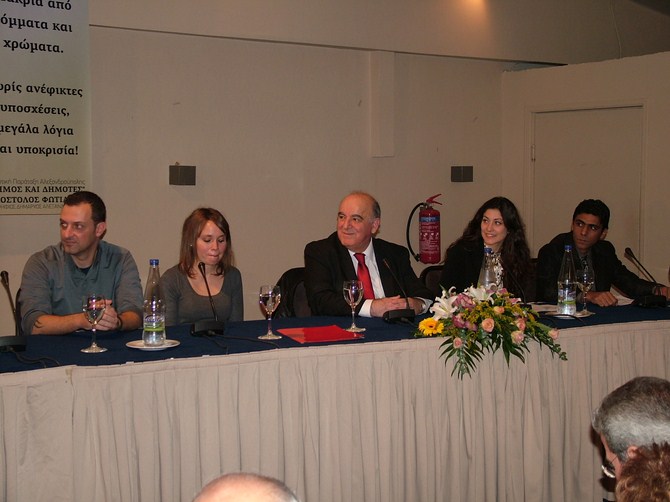This rectangular indoor photograph captures a panel discussion at what appears to be a conference. The backdrop is an unadorned white wall, providing a sharp contrast to the long table adorned with a navy blue top and a white drape skirting that reaches the floor. Five panelists are seated behind the table, each with a microphone and either a water bottle with a glass or a glass of water, suggesting they are preparing to speak. 

On the far left, there is a middle-aged man in a blue shirt, his attention directed to the left. Next to him is a younger woman with long brown hair, dressed in a gray shirt and looking down. The central figure is the oldest panelist, a man in a black business suit and red tie, also looking to the left. To his right is another woman, younger, with black hair, who is wearing a black jacket over a white blouse. On the far right is a man with darker skin, potentially of Indian descent, in a dark suit jacket, similarly looking to the left. 

The table also features a decorative bouquet of fresh flowers towards the center-right, adding a touch of color. Behind the panelists is a sign with what appears to be Russian text. The photograph is taken from the audience's perspective, evidenced by the partial visibility of several audience members' heads in the foreground, attentively listening to the discussion.